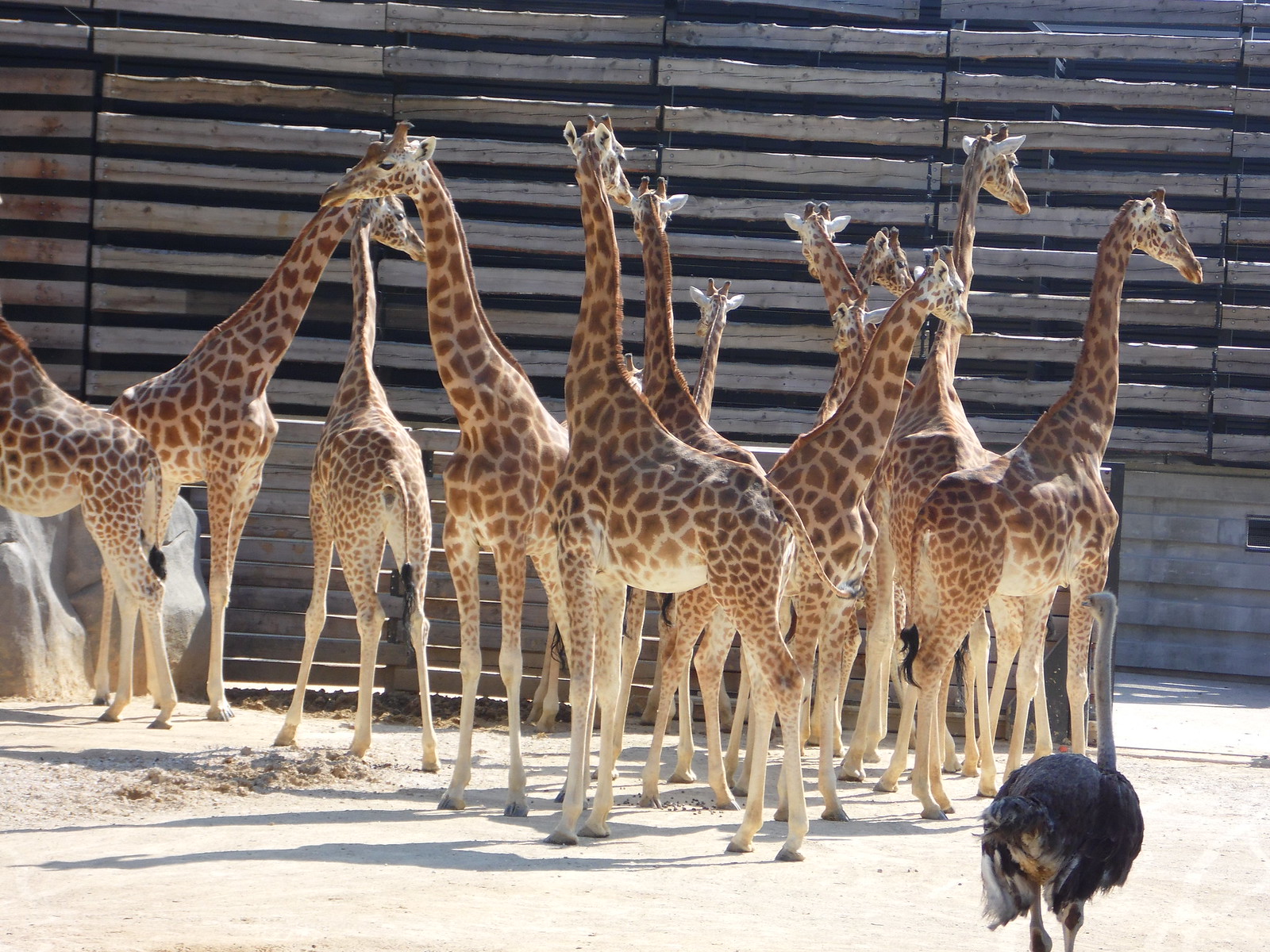In this outdoor photograph likely taken at a zoo, a herd of 10 to 12 giraffes is gathered in front of a tall enclosure made of horizontal timber slats, creating an intricate pattern. The giraffes, all of varying heights but primarily young, showcase light brown bodies adorned with darker reddish-brown spots. They stand on a sandy dirt ground, their long shadows cast clearly beneath them. Some giraffes face the metal-reinforced wooden wall, while others look in various directions, highlighting their majestic necks and elegant stances. In the lower right corner, an ostrich with a striking black back and long white neck gazes towards the giraffes, adding to the scene's dynamic. Partially visible, the ostrich's legs blend into the sandy ground, and a noticeable rock sits at the bottom left, framing the natural ambiance of the enclosure.